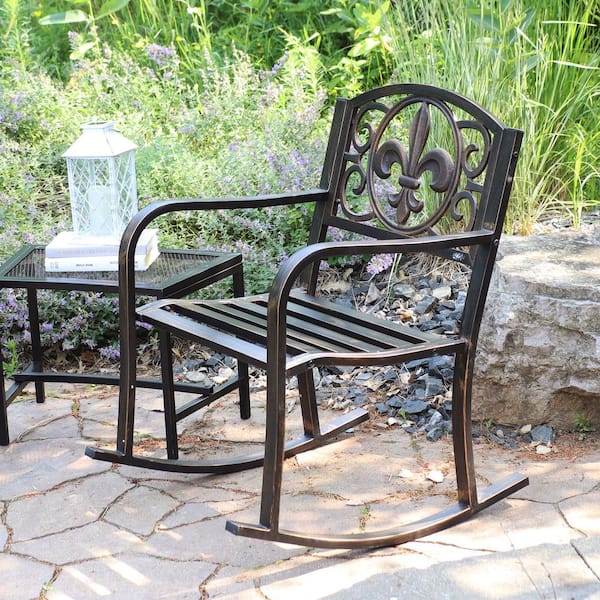This outdoor photograph depicts a bronze rocking chair facing left, situated on a stone patio. The chair, which has a modern design yet evokes a classic feel, features a square-shaped armrest and a large, ornate circular back with a fleur-de-lis design reminiscent of the New Orleans Saints logo. To the right of the chair is a black mesh-topped coffee table with a matching black frame. On the table, a gray book rests atop a white book, and a white lantern is carefully placed on top of them. Encircling the stone patio are vibrant tall pink-lavender wildflowers to the left and lush tall grasses to the right, creating a serene and picturesque setting.